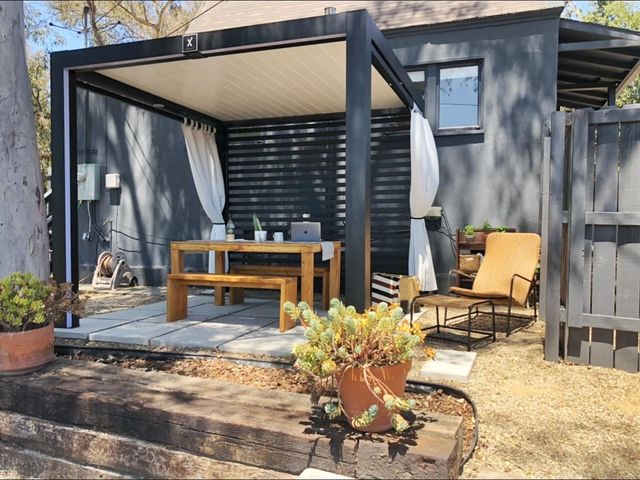In the daytime photo of a back patio attached to a dark gray house, various elements create a harmonious outdoor living space. At the forefront, two potted plants rest on the edge of wooden steps. The first planter, a brown pot, holds a green plant with a brownish one to its right. The second, made of orange clay, houses yellow-gold flowering plants with some buds still closed. A soil bed lined with orange mulch lies in front of these planters. 

The patio features a dark blue gazebo with a white-painted steel roof and white curtains, which are pulled back, presumably to shield from the sun when needed. Underneath the gazebo, a wooden table with a light brown finish is flanked by two matching benches. On the table sits a MacBook laptop and two glasses. 

An orange chair and a cyan-colored fuse box are present on the right and left sides of the scene, respectively. A tall tree stands to the left while an open gray-painted gate is visible on the right. The surrounding grass appears brownish-orange, complementing the earthy tones of the scene. The backdrop includes a window on the right side of the building, adding to the patio's connected and inviting atmosphere.